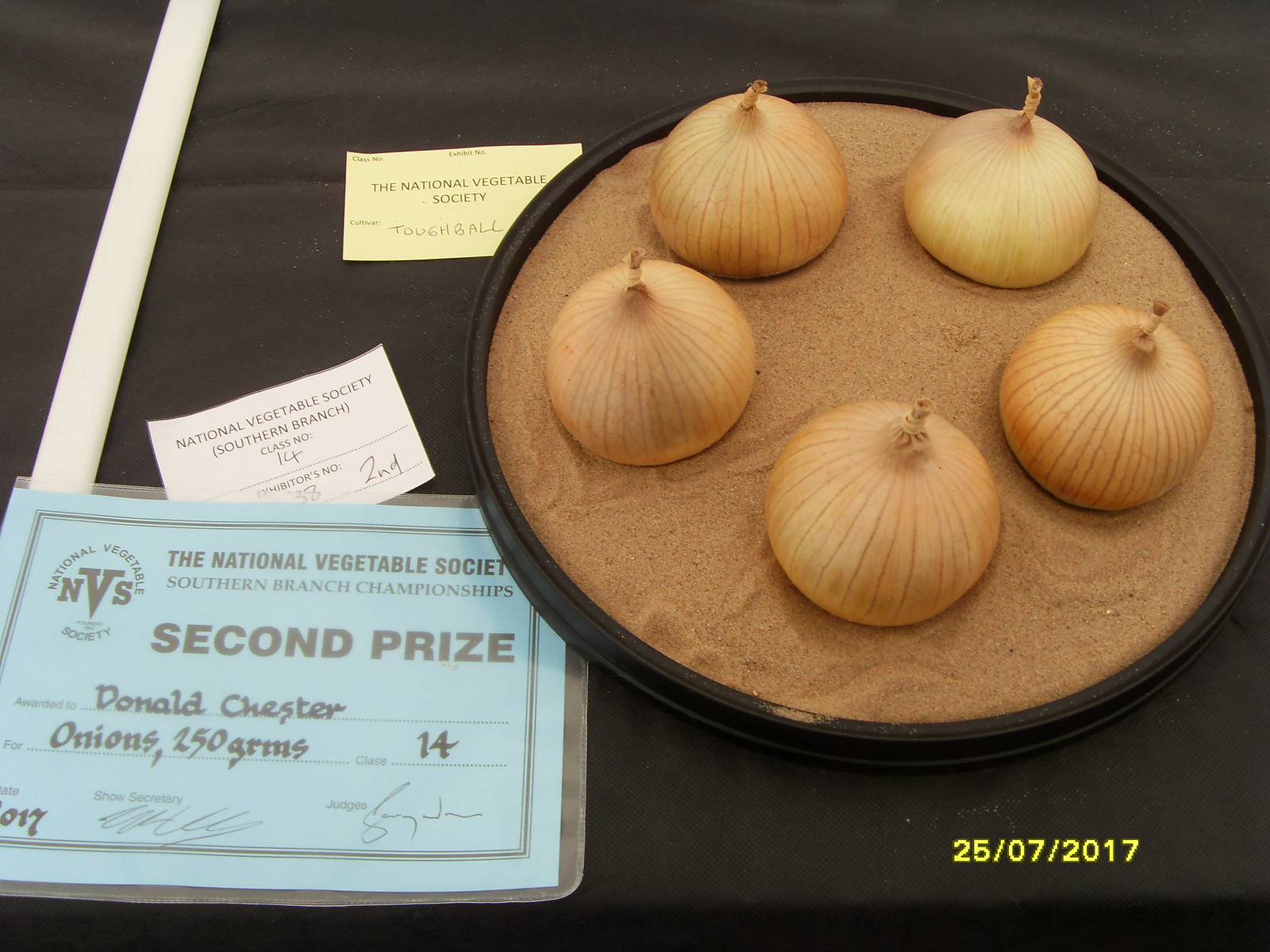The image depicts a vegetable display on a dark-colored table, featuring five meticulously arranged onions on a round wooden platter with a black border, filled with sand. The onions are perfectly round and form a star pattern, positioned evenly. To the left of the platter, a blue laminated card from the National Vegetable Society Southern Branch Championships announces that Donald Chester won second prize for onions weighing 250 grams in class 14. The card bears the signatures of officials. Above this, another card, identifies the cultivar as "Toughball", accompanied by further details. The image is dated 25-07-2017, prominently displayed in yellow in the lower right corner.